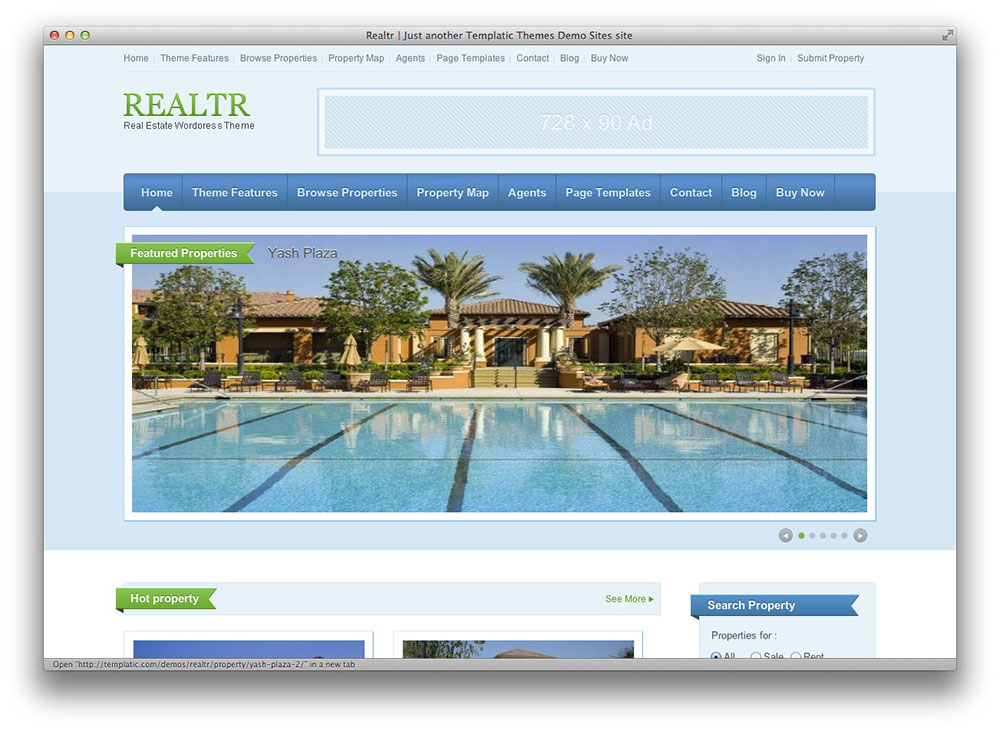**Website Screenshot of R-E-A-L-T-R for Real Estate**

The screenshot captures the homepage of the R-E-A-L-T-R website, a real estate WordPress theme. The top section of the page is set against a white background with black text, listing the main menu options horizontally. These options include: Home, Theme Features, Browse Properties, Property Map, Agents, Page Templates, Contact, Blog, and Buy Now. To the right of the menu, there are additional options for Sign-In and Submit Property.

Occupying the topmost portion of the page is an empty ad space designated for a 728 by 90 advertisement. Adjacent to this ad space on the left is the website's logo, displayed as "R-E-A-L-T-R" in green, using the Times New Roman font. Beneath the logo, the text "Real Estate WordPress Theme" is present.

Below this section, a blue navigation bar mirrors the initial menu options in white text against the blue background, ensuring easy access to primary site features. 

The main content area prominently showcases a large photograph that takes up nearly the entire width of the webpage and about half of its height. The featured property in the image is titled "Yash Plaza." The photograph depicts a serene setting with a swimming pool in the foreground, which occupies the lower portion of the image, and a tan-colored house in the background. The scene hints at a southern locality, complete with palm trees and patio furniture surrounding the pool.

Directly below this feature photo is another banner labeled "Hot Property," accompanied by a link labeled "See More" and a "Search Property" function. The remainder of the webpage is not visible in the screenshot.